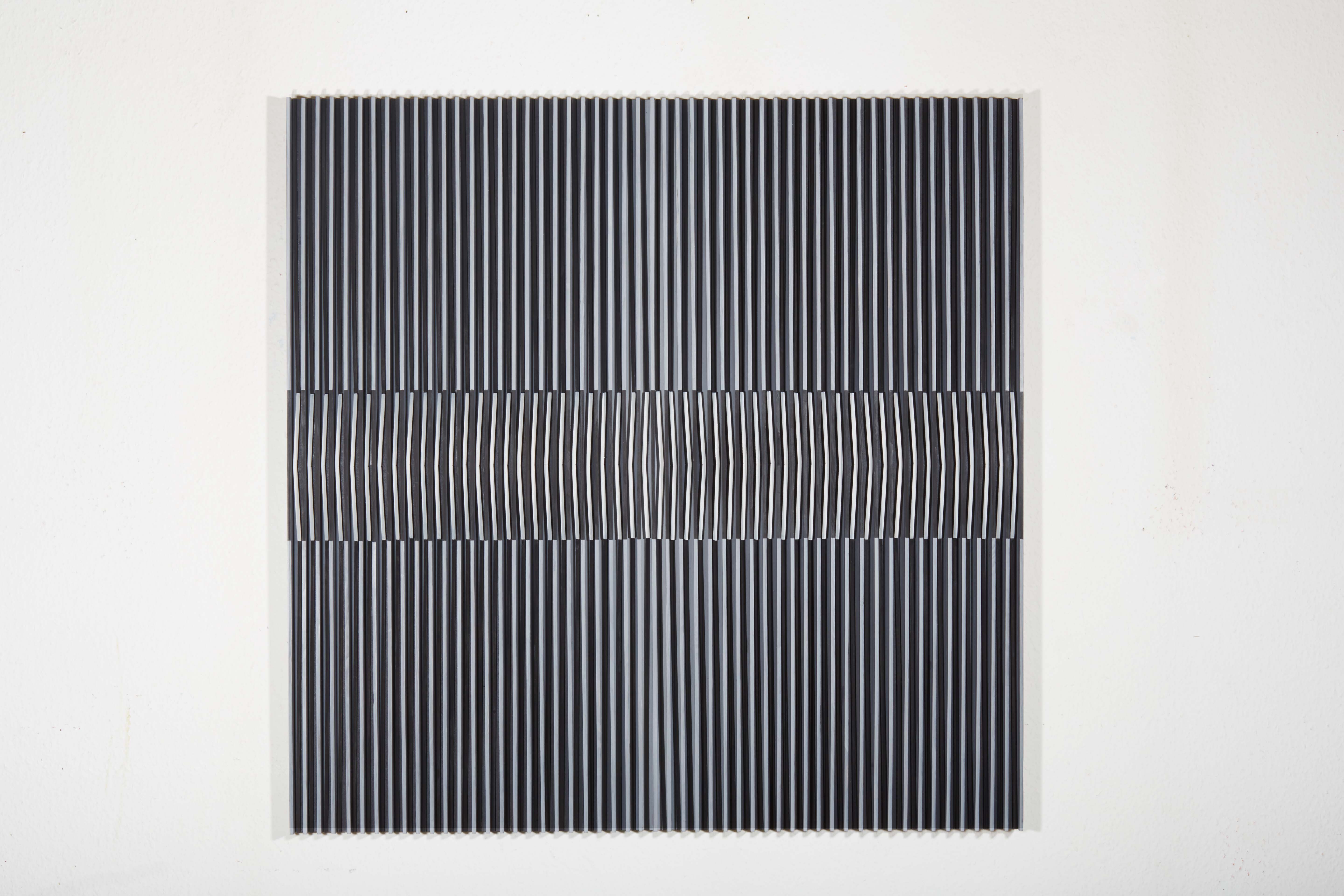The photograph captures a captivating piece of artwork that initially gives the impression of an air conditioning vent but reveals more complexity upon closer inspection. The art is rectangular and consists of a series of thin vertical black and white lines. The black background is segmented into three sections, with a prominent distortion in the middle. In the center, the white lines are misaligned compared to the top and bottom sections, creating a 3D illusion that draws the viewer in. This central band curves outward, forming a diamond-like shape that enhances the sense of depth. The piece is bordered by plain white on all sides, contrasting sharply with the intricate pattern within. The entire composition is set against an off-white wall, amplifying its visual impact and giving a striking, almost bizarre, yet mesmerizing effect.